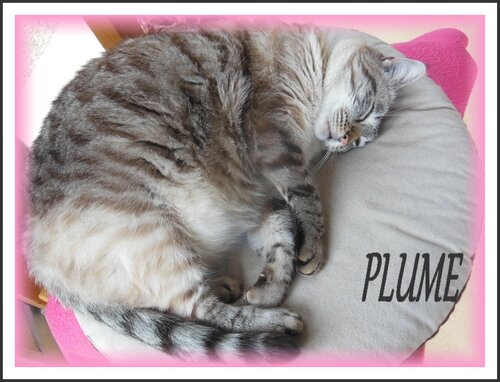A fluffy, overweight tabby cat named Plume is peacefully napping on a perfectly circular, light gray pillow that takes up 30% of the image. Plume's eyes are closed, his body is slightly curled up with feet tucked under, and his striped tail rests along his bottom leg. The cat's fur is an intricate mix of gray, white, black, and beige patches, with significant dark brown stripes and white whiskers. The inside of his ears are white, further adding to his multicolored appearance. The background of the image is framed by a pink and white border, while the cat's name "Plume" is clearly written in dark gray text on the bottom right corner. The overall scene exudes a sense of coziness and contentment, with Plume filling up 70% of the image, comfortably lounging as if without a care in the world.